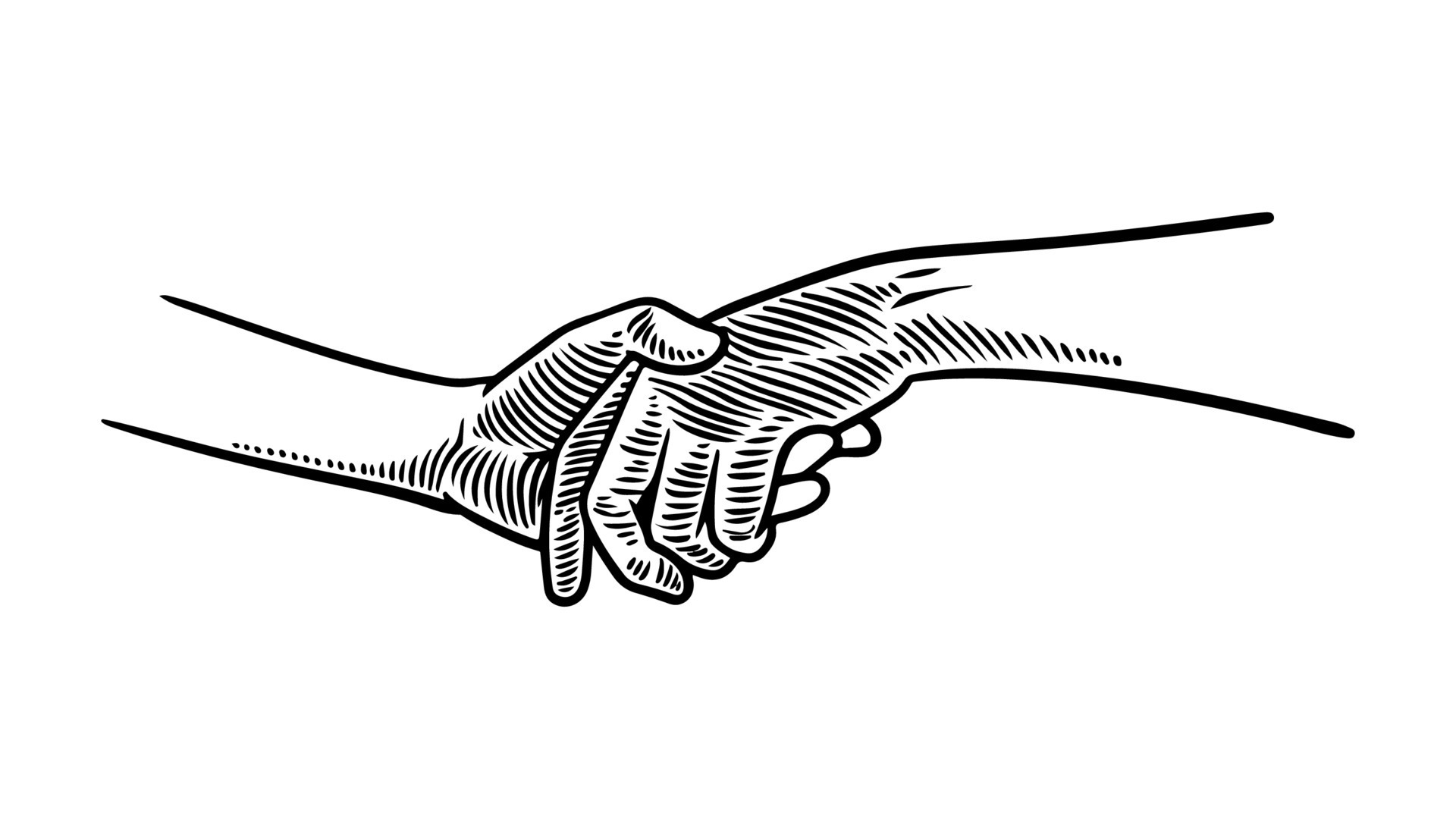This black and white illustration depicts two forearms extending from the left and right sides of the image, meeting in a handshake at the center. Created with intricate black pen lines, the artwork leans towards a woodcut style. The forearms are highlighted in stark white, contrasting with the hands which are darkened through detailed line shading and cross-hatching. The clasping hands—that suggest a limp grip from one person and a firm grip from the other—are the central focus, with their contours and finger joints emphasized by the dense line work. The illustration, devoid of any boundary, features a plain white background, further accentuating the simplicity and directness of the handshake as the primary subject.